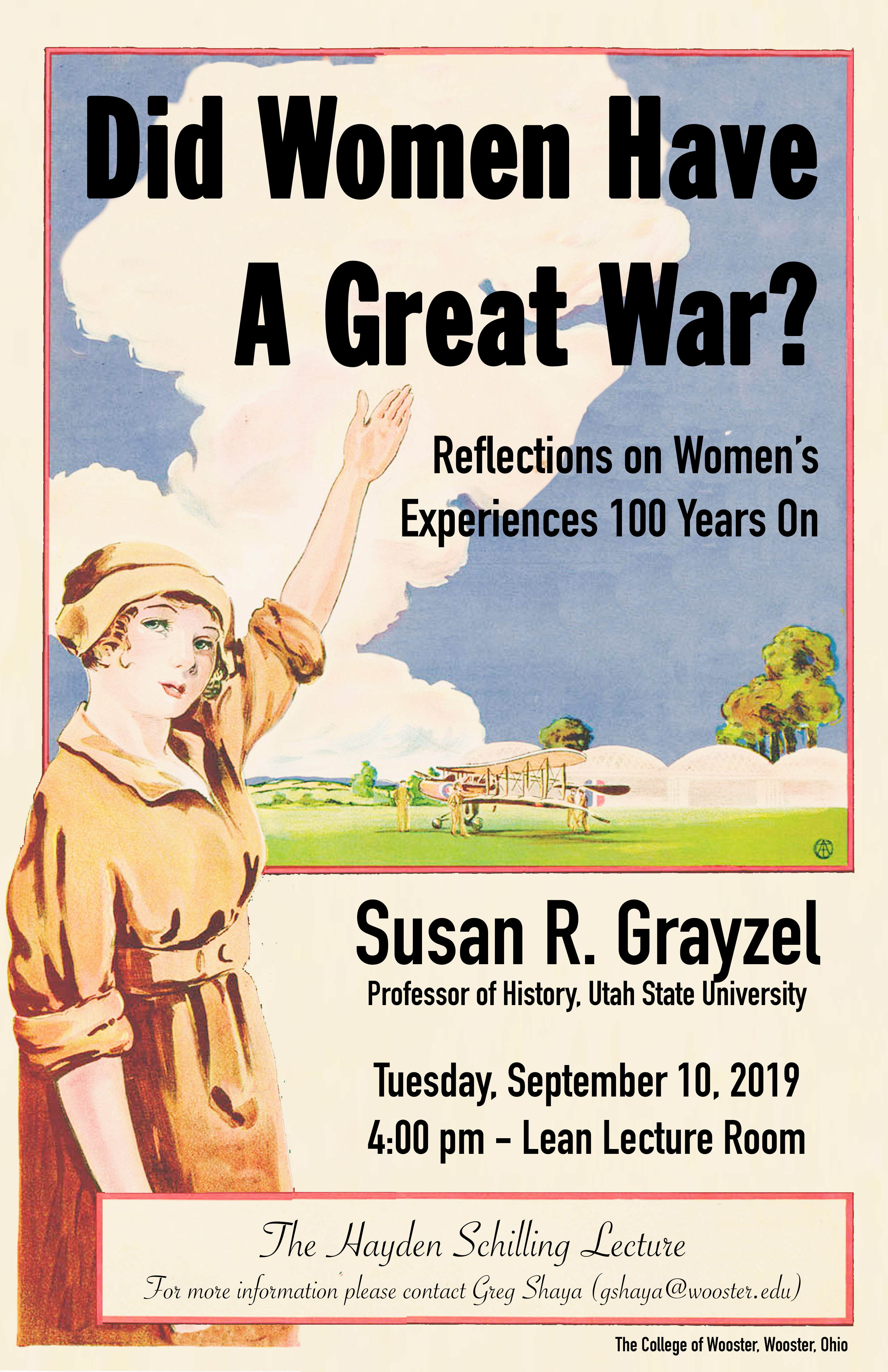This 2019 poster advertises a lecture on a light yellow background with a blue sky and white cloud design at the top, boldly asking in black text, "Did Women Have a Great War? Reflections on Women's Experiences 100 Years On." In the bottom left corner, a woman with light yellow hat, very white pinkish skin, and green eyes stands, one arm raised, wearing a heavy orange coat with a belt. Centrally featured is an early yellow wooden airplane facing left, set against a backdrop of trees and white mountains. Below the image, it reads: "Susan R. Grazel, Professor of History, Utah State University," followed by "Tuesday, September 10, 2019, 4 p.m., Lean Lecture Room." Enclosed in a rectangle, it notes, "The Hayden Schilling Lecture," and provides contact information: "For more information, please contact Greg Shia at gshia@wooster.edu." The very bottom right corner states: "The College of Wooster, Wooster, Ohio."